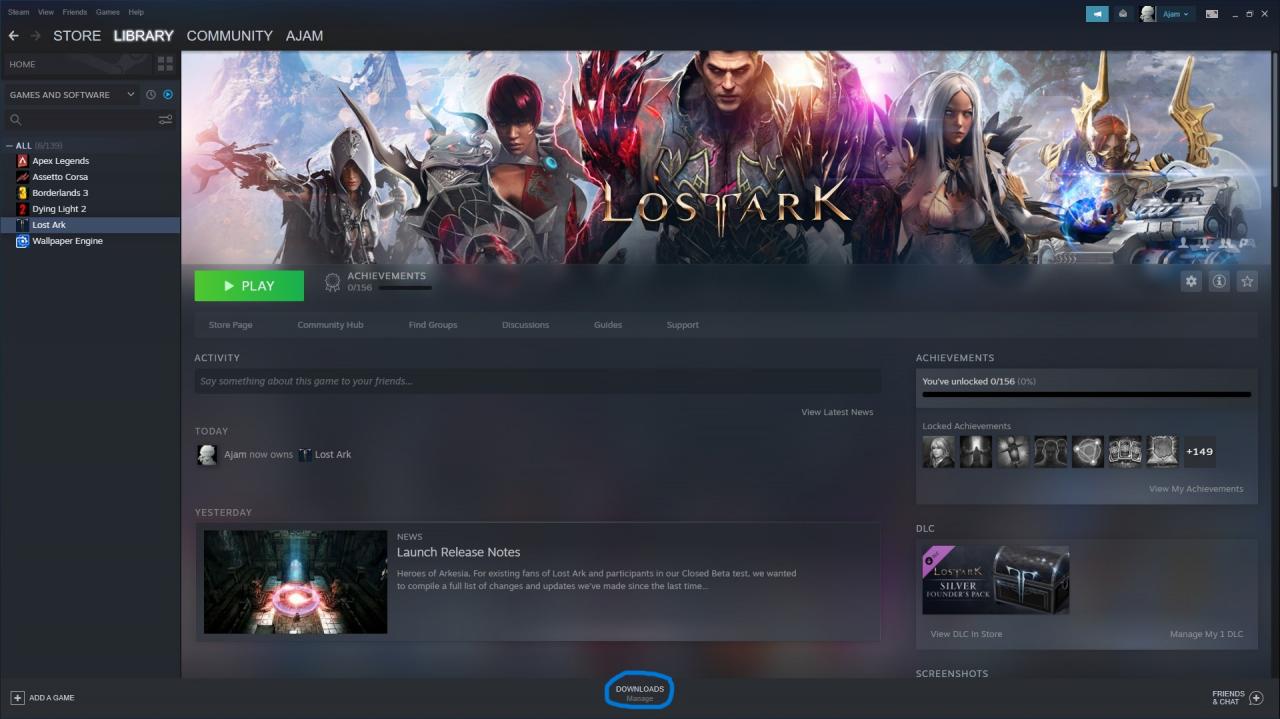The image depicts a vibrant and action-packed scene from the game "Lost Ark." At the center of the image, a formidable figure clad in elaborate armor and equipped with menacing claw hands stands resolutely. Flanking him are two women, one on each side; their expressions and attire hint at their significance in the story. To the left of the woman on his left, a mysterious hooded man adds an element of intrigue and danger. Positioned to the right of the woman on his right, a character carrying a large gear on his back and armed with a gun conveys readiness for battle.

The bottom of the image displays the text "Launch Release Notes." Below this, a glowing purple circle illuminates a hallway, likely indicating a portal or significant in-game location. To the right of this, a blue circle highlights "Downloads Managed," suggesting an interface or functionality within the game or gaming platform. Accompanying these elements are screenshots on the right, showing dynamic in-game scenarios, a chat interface where friends are active, and another game emblem featuring a treasure chest, symbolizing adventure and rewards. This detailed depiction captures the essence of "Lost Ark," blending character dynamics and game mechanics into an engaging visual narrative.